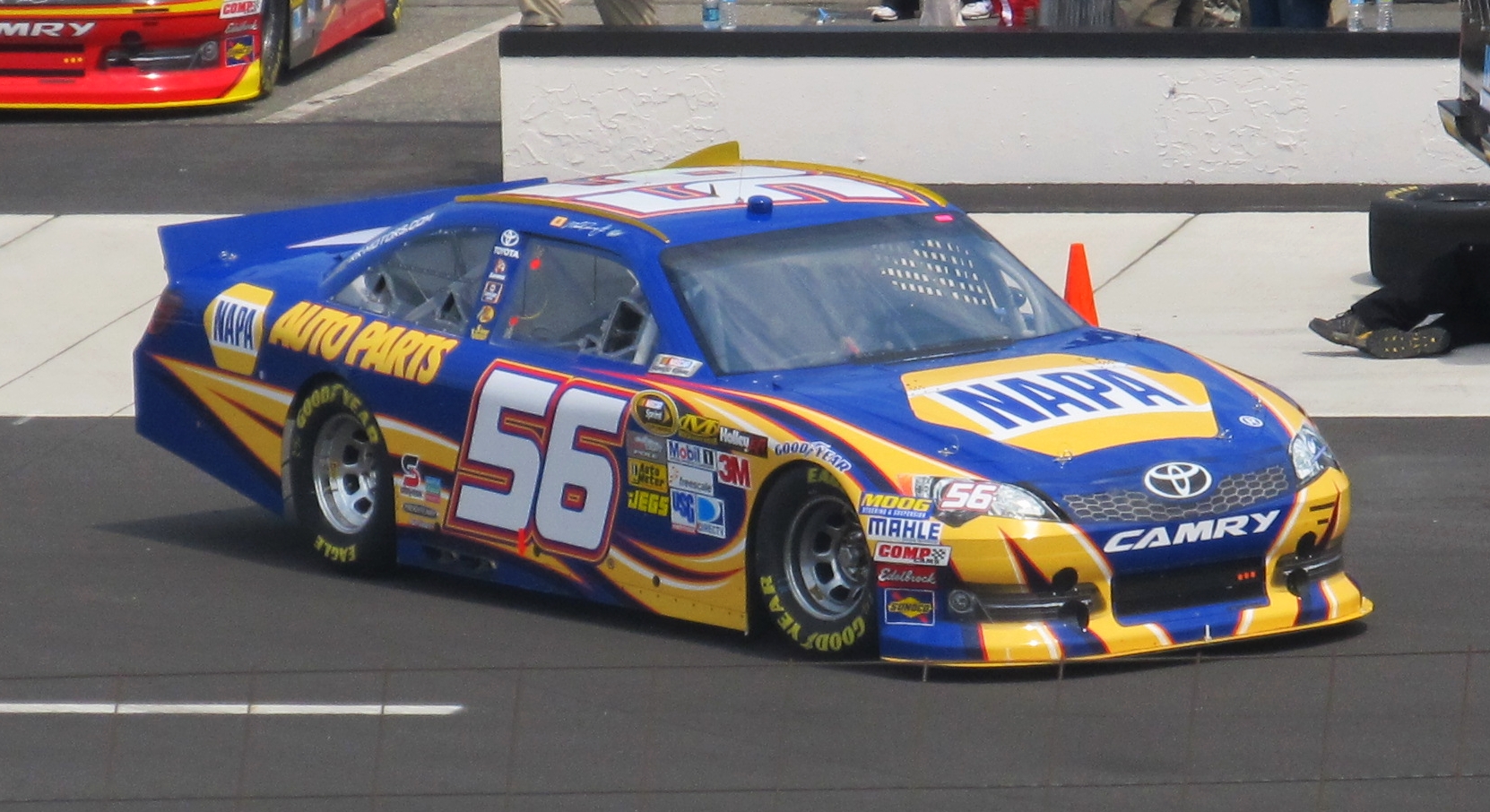This is a detailed color photograph of a blue race car, captured mostly from the side as it speeds along a black asphalt racetrack. The car is adorned with intricate blue, white, and yellow graphics, including a notable red-outlined flame design. The bold, white number "56" and the prominent "Napa Auto Parts" text in yellow and blue are easily readable along its side, accompanied by various smaller sponsor logos such as Mobile, 3M, and others. These logos extend towards the front bumper, which displays the word "Camry" in white lettering, underlined by the unmistakable Toyota logo. The hood prominently features "Napa" in blue lettering against a white and yellow backdrop. The background includes a white wall, a barely visible red race car in the upper left-hand corner, and a glimpse of pavement markings. In the upper right-hand corner, the feet of a person working underneath a car can be spotted.